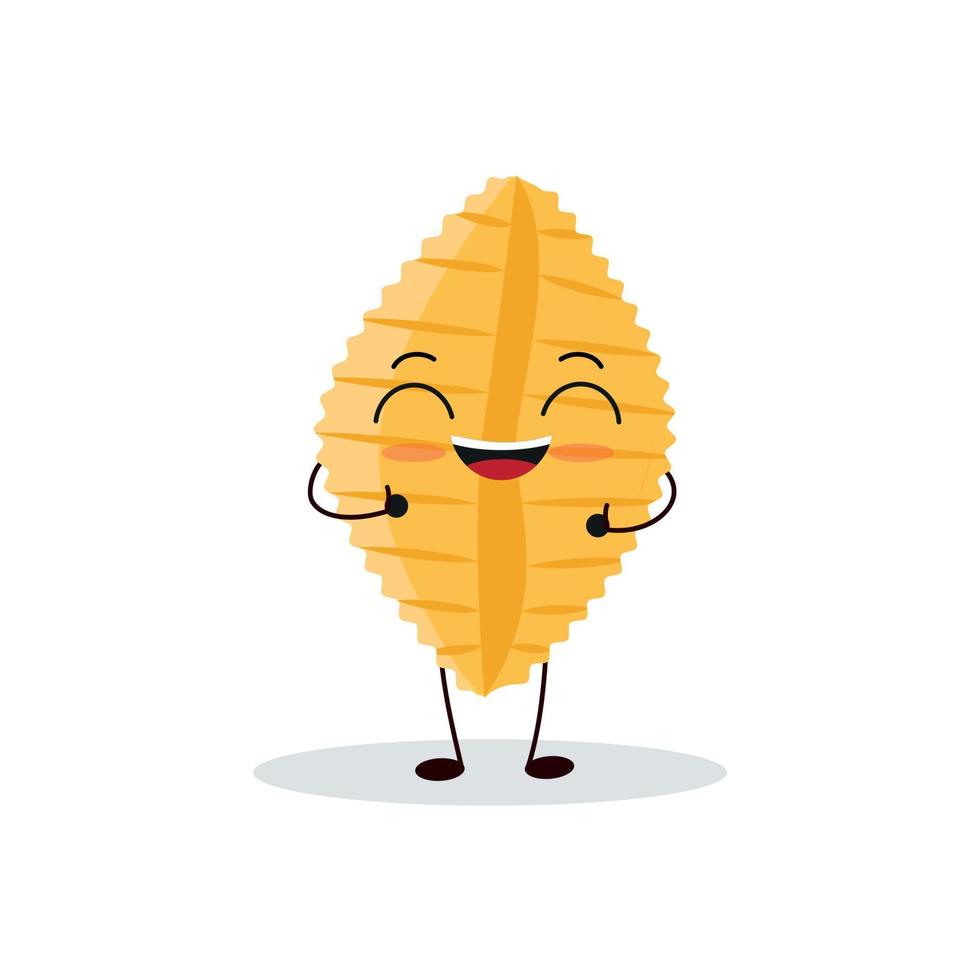The image is a computer-generated illustration resembling a character made from a pasta shell, particularly similar to a conch or stuffed shell. The character is predominantly orange and beige, featuring a simple yet expressive cartoon face. It has semicircle eyebrows, closed eyes shaped like upside-down U's, and a wide open-mouth smile with a red tongue visible inside, akin to a half-moon. Blushing marks, depicted as small pink spots, can be seen on its cheeks.

The character possesses minimalistic arms and legs, drawn as thin black lines. The arms curve forward and give a thumbs-up sign, while the legs, looking like music notes or stick figures, extend downward. It stands on a white background with a light gray oval shadow beneath it, grounding the character in the scene.

The shell itself has jagged edges along its sides and a noticeable stripe running down the middle, enhancing its likeness to an actual pasta shell. This cheerful, kid-like cartoon image combines simplified lines and shapes to create a delightful and whimsical character.